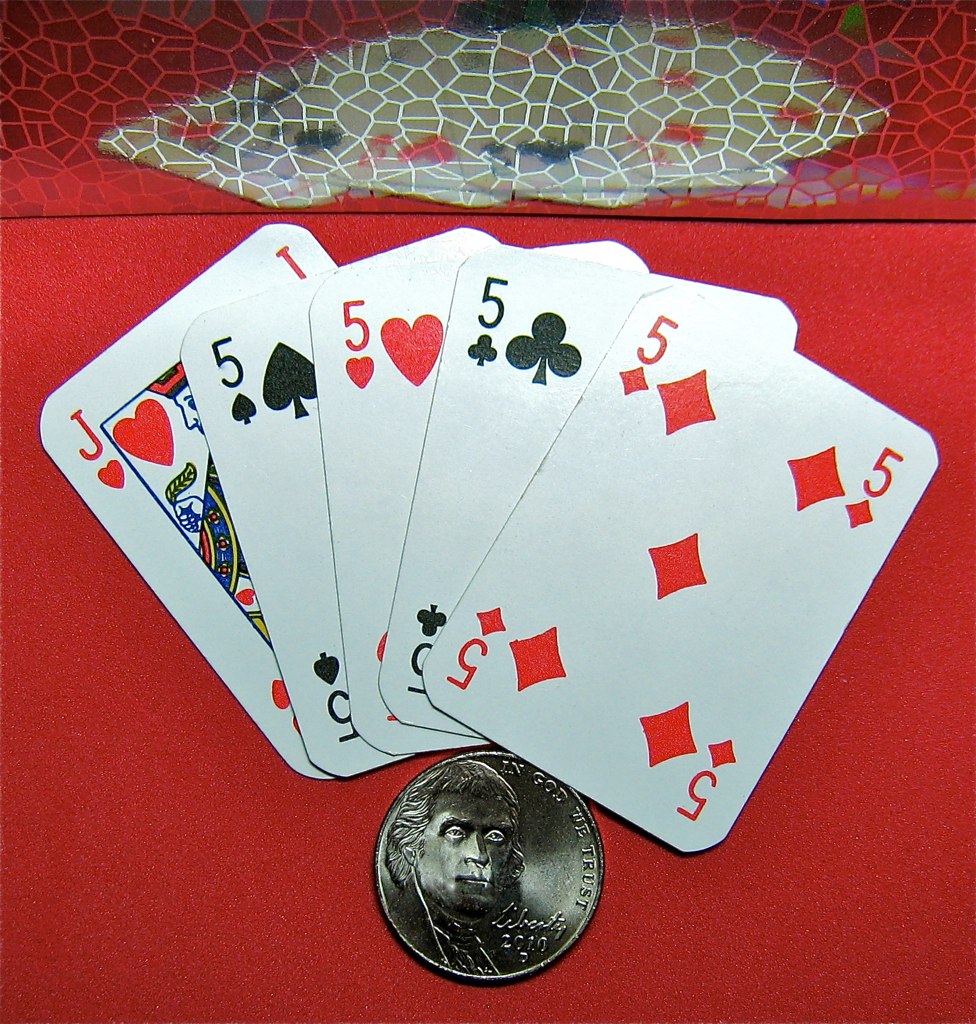A close-up photograph depicts a fan of five playing cards lying on a red cloth tablecloth. The cards include four 5s and one Jack. A quarter, dated 2010 and displaying the inscriptions "In God We Trust" and "Liberty," touches one of the cards. Behind the cards, a texture-rich, shiny red surface with a pebble-like pattern is visible. Slightly overlapping this surface is an oblong, pointy object adorned with blue and red spots.